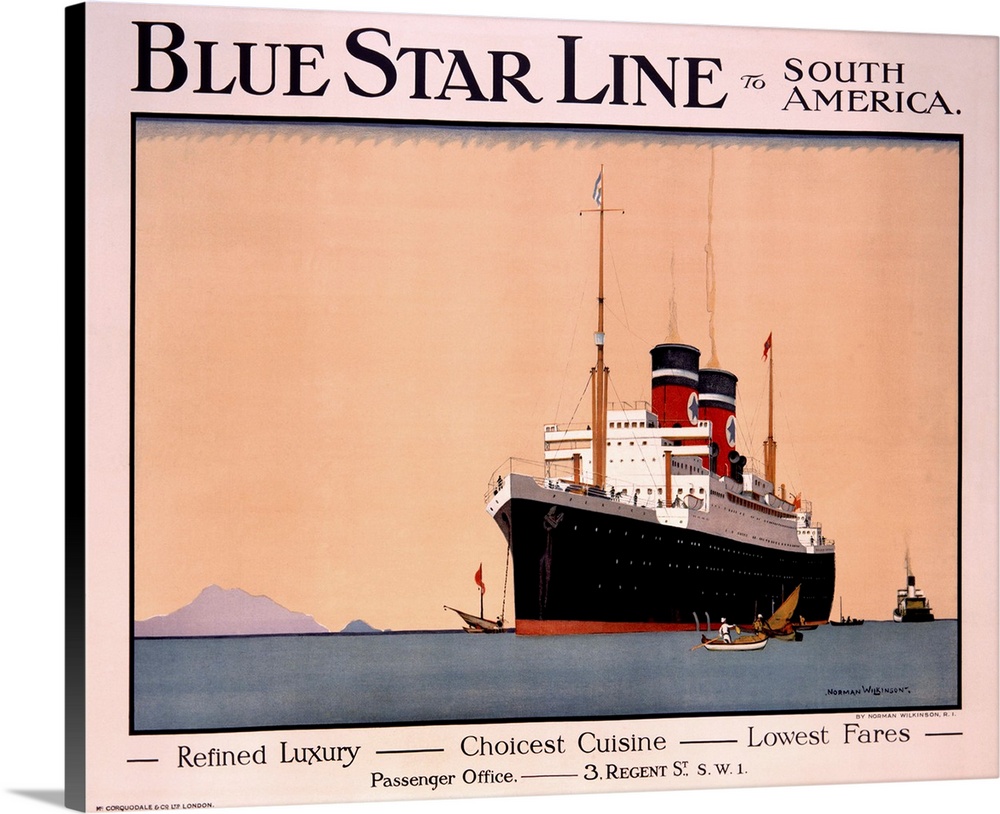Caption: 

This canvas artwork portrays the vintage cover of a box, possibly used for promotional purposes by a historical shipping line. At the top, in a large, dark font, it reads "Blue Star Line". Beneath this, in a thinner, smaller font, the text "To South America" is inscribed. The central image features a grand vessel pointing towards the lower left corner, with the water beneath rippling gently. Surrounding the large vessel, small canoes add a contrasting element of scale and simplicity. Below the image, the promotional tagline "Refined Luxury, Choicest Cuisine, Lowest Fares" is displayed, emphasizing the high standards and affordability of the Blue Star Line's services.